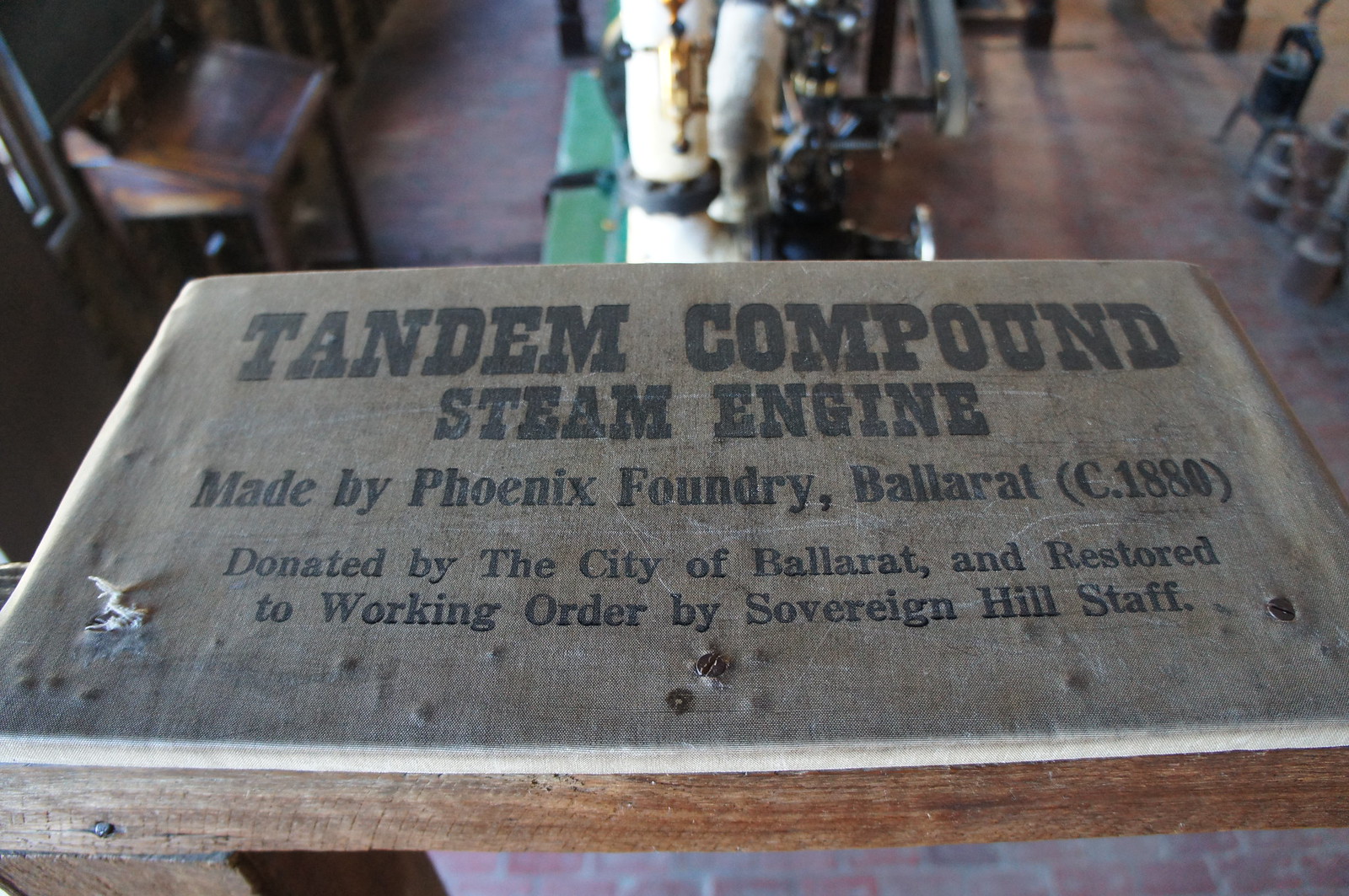The photograph features an aged wooden sign, lying flat on a wooden surface, with black text that reads: "Tandem Compound Steam Engine, made by Phoenix Foundry, Ballarat, circa 1880. Donated by the City of Ballarat and restored to working order by Sovereign Hill Staff." The sign, which has a weathered appearance, is set against the backdrop of what seems to be a vintage workshop area. In the background, partially visible, is likely the steam engine the sign refers to, with some indistinct wooden objects, possibly an old desk, and other items scattered around. The floor appears to be wooden, suggesting a historical setting. The overall image, though vivid, gives a sense of antiquity, blending elements of the past with a preserved, restored look, making it hard to pinpoint the photograph's exact age.